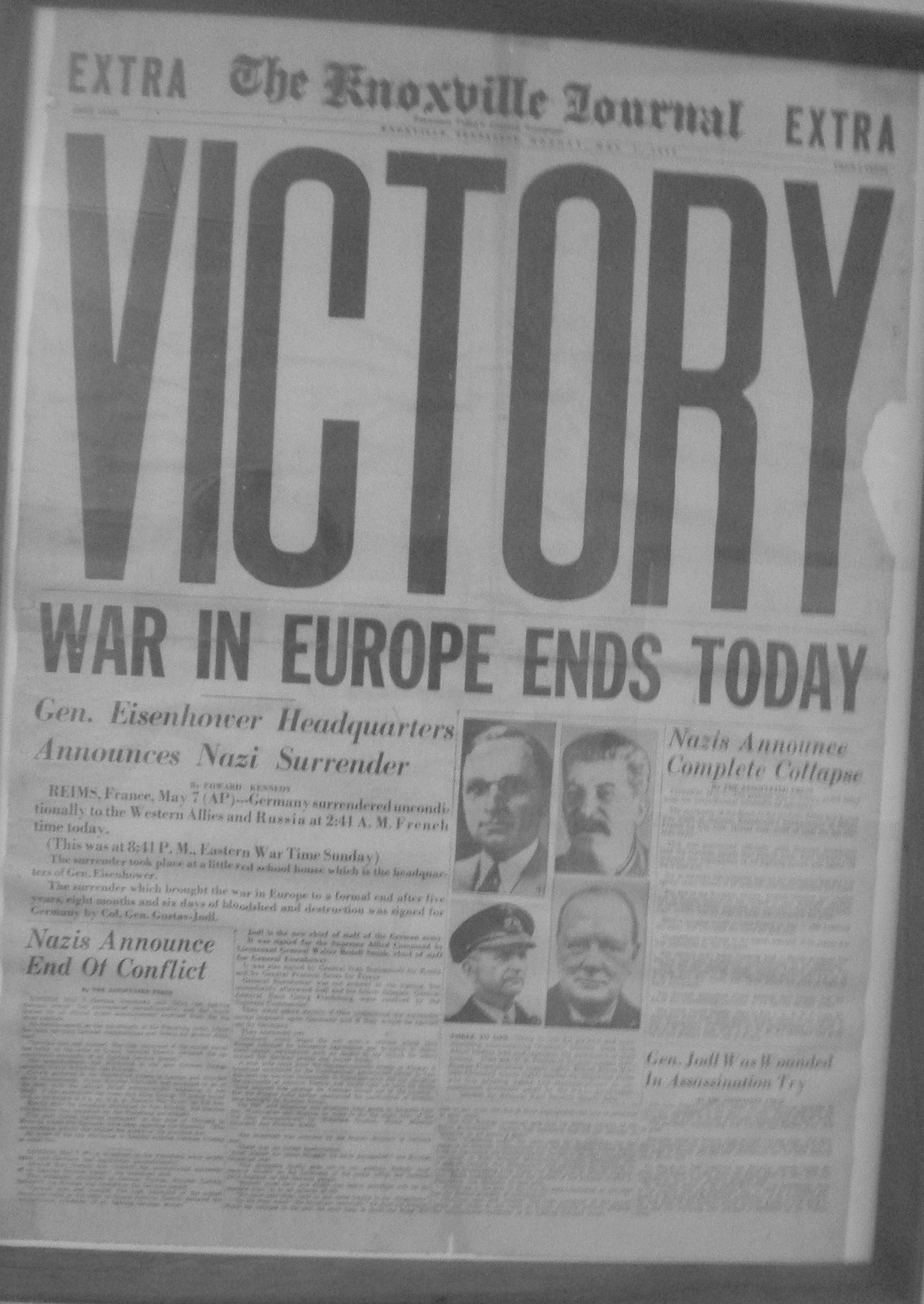This is a photo of the front page of the Knoxville Journal entitled "Extra." In large, bold letters at the top, the word "Victory" dominates the page. Beneath that, the headline reads, "War in Europe Ends Today," with a sub-headline stating, "General Eisenhower Headquarters Announces Nazi Surrender." The dateline reveals: "R.E.I.M.S. France, May 7th, AP - Germany surrendered unconditionally to the Western Allies and Russia at 2:41 a.m. French time today. This was at 8:41 p.m. Eastern Wartime Sunday." Other headlines include "Nazis Announce End of Conflict" and "Nazis Announce Complete Collapse." Another headline reports, "General Joel W.E.S. Wounded in Assassination Try."

The center of the front page features four photographs: Harry Truman, Joseph Stalin, Winston Churchill, and General De Gaulle. The overall aesthetic of the image is in faded gray, characteristic of an old black-and-white newspaper. The smaller print is unreadable due to the resolution. This momentous edition likely dates from May 7, 1945, marking the conclusion of World War II in Europe.